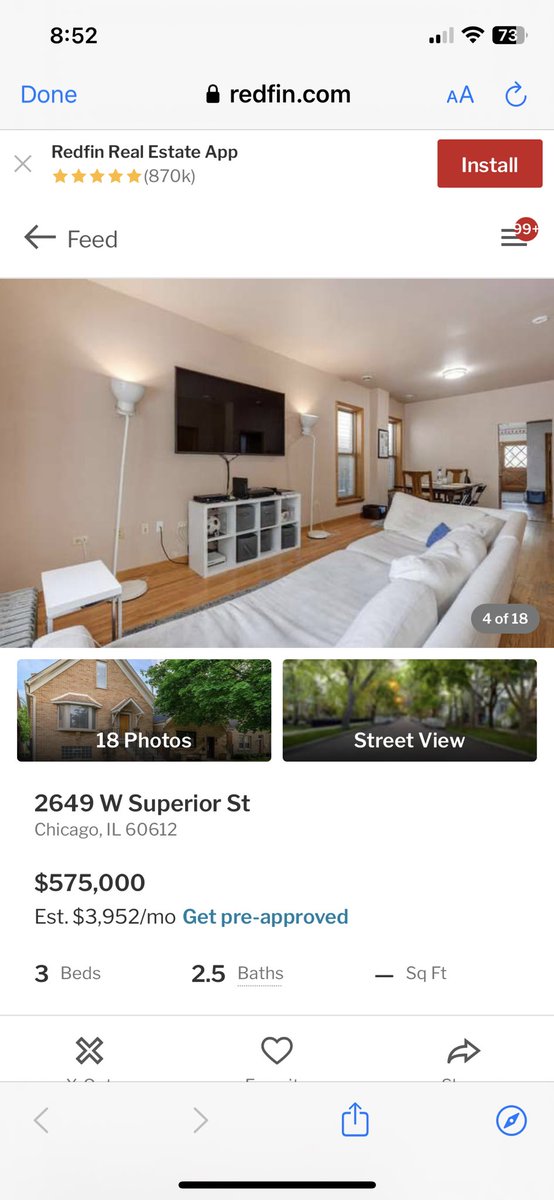This image is a cropped mobile screenshot of a real estate listing on Redfin.com. At the top of the screenshot, there is a black lock icon alongside the text "Redfin.com." To the left, a blue "Done" button is visible, while the right side features a font icon and a refresh icon. The background of the image is white.

At the top of the listing, a small pop-up with an "X" on the left side allows for closing the pop-up. To the right of the "X," the text "Redfin Real Estate App" is displayed, followed by a rating of 5 stars based on 870,000 reviews. Next to the reviews, there is a red "Install" button.

Beneath this pop-up, there is a "Feed" label with thumbnails of properties displayed below. The main large thumbnail, occupying the central part of the image, showcases a living room scene with a small label indicating "4 of 18," signifying that this is the fourth photo in a carousel of eighteen images. Below this large thumbnail, there are two smaller thumbnails: one depicting the exterior of the house marked with "19 photos" and another showing a street view labeled "Street View."

Further down, the screenshot displays the property address followed by the listing price. Beneath the price, the text "Estimated Monthly Payment" is shown, with an option to get pre-approval highlighted in blue writing.